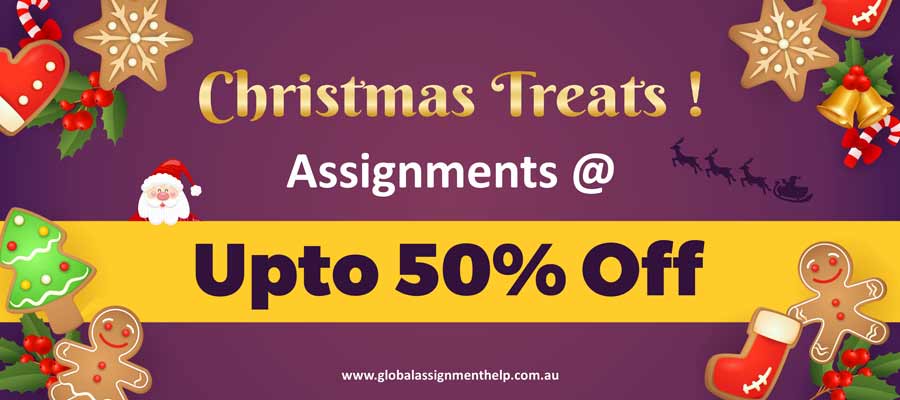Screenshot caption:

"Christmas Treats" is displayed prominently in eye-catching, bubble letters with a gradient effect transitioning from gold at the top to beige in the middle and back to gold at the bottom. Positioned near the upper portion of the image, the title sets a festive tone. Below the title, the text "assignments at www.globalassignmenthelp.com.au" is written in white.

Centrally, closer to the bottom, a bold yellow rectangle announces a special offer, stating "up to 50% off" in striking purple letters. The entire background of the image is a dynamic gradient of purple, which is lighter in the middle and gradually deepens to darker purple towards the edges.

Adding to the festive theme, an assortment of Christmas-themed graphics decorates the corners of the image. These include an array of cookies shaped like a star, a mitten, a Christmas tree, a gingerbread man, and a stocking. Additional festive elements, such as a candy cane adorned with a red bow, a Christmas wreath, bells, and an image of Santa Claus, enhance the holiday cheer.